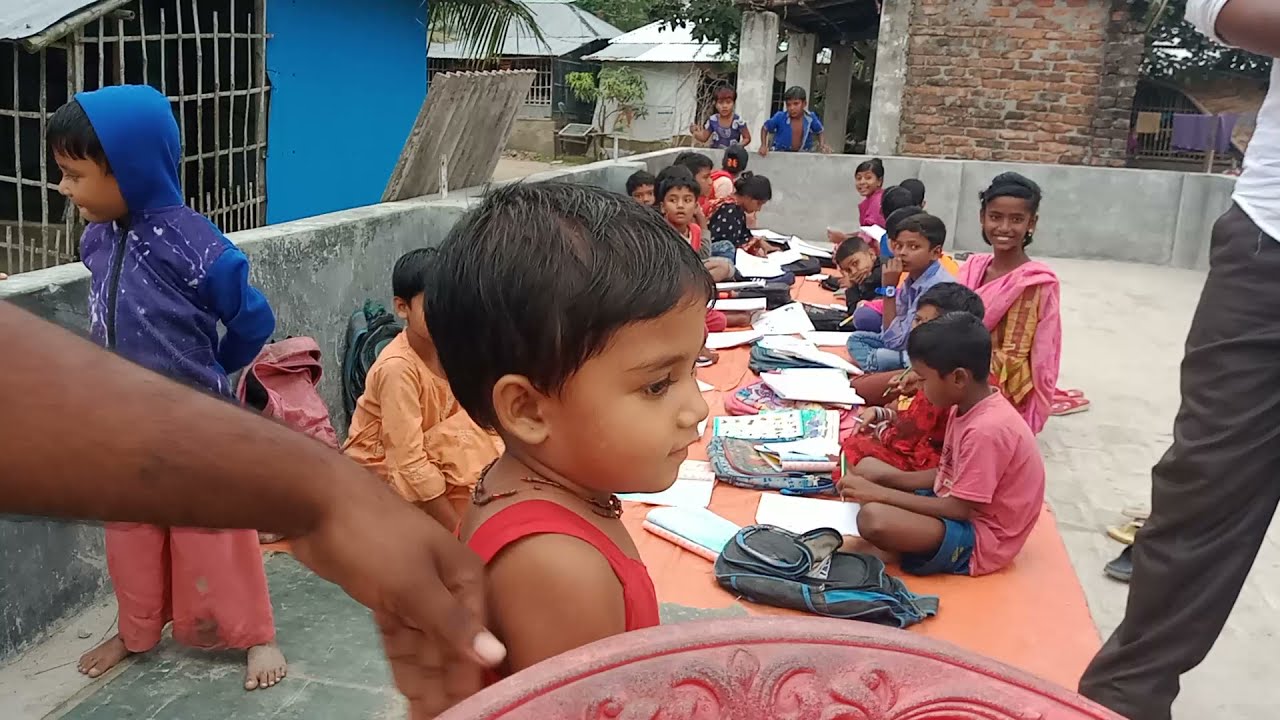This image captures an outdoor educational activity taking place on a concrete patio area surrounded by a barrier wall and overlooking a village with jungle-style foliage. The scene is bustling with approximately two dozen children, likely between the ages of 8 and 12, suggesting a school setting in an Asian country, possibly India. They are seated cross-legged on a long, pink mat that has been spread out on the ground. Each of the children is engaged with school supplies laid out before them, including books, pencils, and backpacks, suggesting they are focused on some kind of learning or homework.

The children are dressed in a variety of clothing, ranging from t-shirts and shorts to long-sleeved jackets, indicating a casual, possibly warm-weather setting. Among them is one notable young girl with long black hair tied back in an elaborate style, wearing earrings and a pink shawl, who might be slightly older or playing a supervisory role. The scene also includes adults; notably, a man's leg is visible to the right, and on the left, an adult's hand is gently touching a young boy in the foreground, who is dressed in a pink tank top.

The background reveals a slightly rundown village area visible over the concrete barrier, with other buildings and people in sight. There is sand scattered on the patio and a pair of flip-flops. In the forefront of the image, there's a young boy in a red tank top and bead necklace, looking to the right, while another boy in a blue hoodie and baggy red pants is on the left, sitting barefoot.